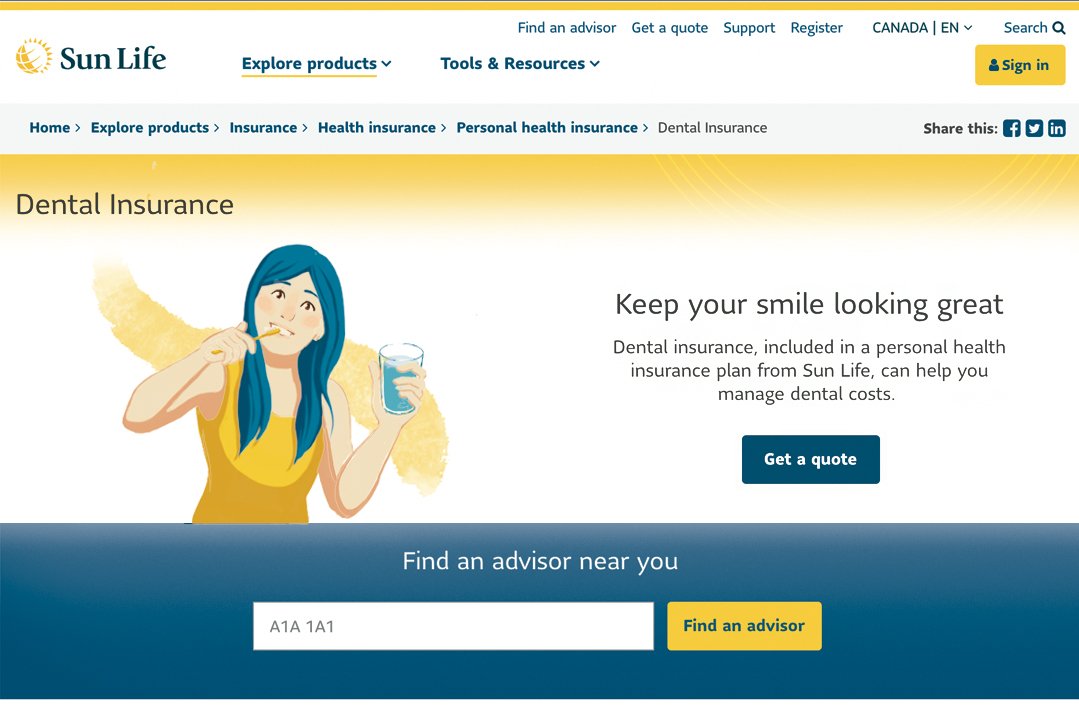The image is a detailed screenshot of the Sun Life web page dedicated to dental insurance. The top navigation bar features various options, including "Find an Advisor," "Get a Quote," "Support," and "Register." There is also an option to change the region from "Canada" to "Canada English" and a drop-down menu for switching the website's language to French. Additionally, a magnifying glass icon for search functionality and the Sun Life logo are present.

Beneath the primary navigation, there are more headings in an aqua blue font, such as "Explore Products" and "Tools and Resources," each with drop-down menus. A prominent yellow or gold button with an icon of a person and the text “Sign In” in aqua blue is also displayed.

Further down, a breadcrumb trail shows the navigation path: Home > Explore Products > Insurance > Health Insurance > Personal Health Insurance > Dental Insurance. The text "Dental Insurance" is highlighted in gray, indicating the current page. To the right, the image offers social media sharing icons for Facebook, LinkedIn, and Twitter.

A yellow bar at the top of the main content area reads "Dental Insurance," accompanied by an illustration of a girl with blue hair brushing her teeth with a blue toothbrush in her right hand and holding a blue drink in her left hand, likely representing water. She is wearing a yellow dress, and behind her is a yellow splash design. The text next to her reads: "Keep your smile looking great. Dental insurance included in a personal health insurance plan from Sun Life can help you manage dental costs."

Below this section, there is a dark blue button with white text saying "Get a Quote." At the bottom of the screenshot, there is a dark blue rectangle with white text that says "Find an advisor near you," and an input field labeled "a1a1a1," followed by a yellow button with blue text stating "Find an Advisor."